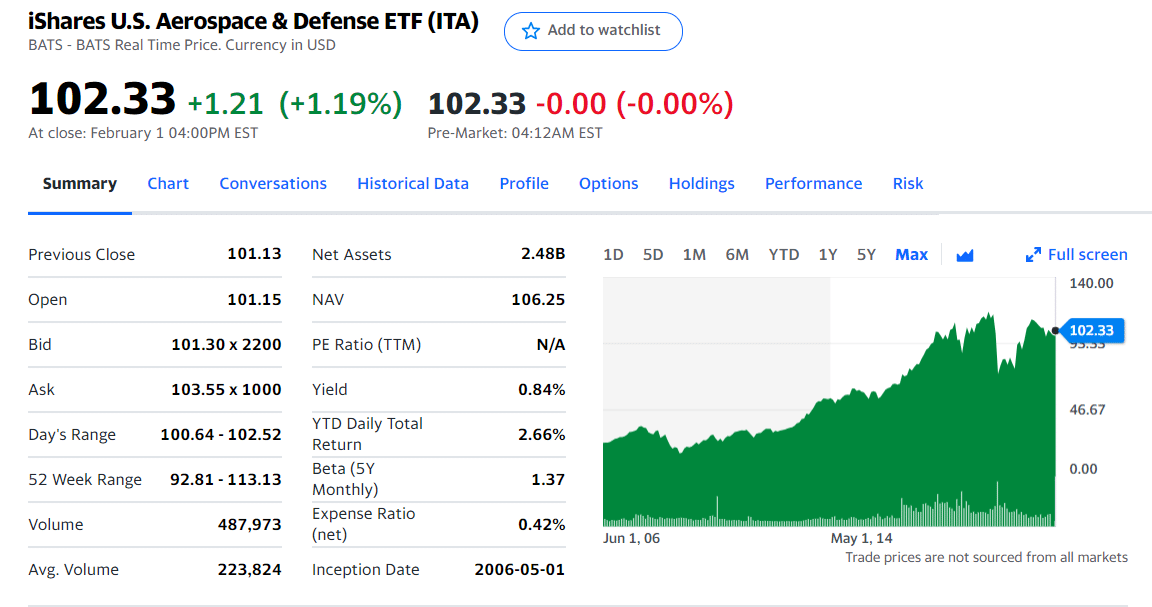This is a detailed analysis of the iShares U.S. Aerospace & Defense ETF (ITA) based on a summary report.

### iShares U.S. Aerospace & Defense ETF (ITA) Overview

- **Current Price:** $102.33 (an increase of $1.21, equivalent to +1.19%)
- **Previous Close:** $101.13
- **Opening Price:** $101.5
- **Bid:** $101.30
- **Net Asset Value (NAV):** $102.33 (unchanged, 0.00%)

### Summary
The iShares U.S. Aerospace & Defense ETF is showing mild positive movement today with a current price of $102.33, reflecting a rise of $1.21 or 1.19% from the previous close. Key details include a bid price of $101.30 and an opening price of $101.5.

### Sections Included in the Report
- **Summary Chart:** Provides a visual representation of the ETF's performance.
- **Conversations:** Discussion and opinions on the ETF.
- **Historical Data:** Analysis of past performance and trends.
- **Profile:** Information about the ETF’s composition and objectives.
- **Options:** Insight into available trading options.
- **Holdings:** Breakdown of the assets held within the ETF.
- **Performance:** Analysis of the ETF's returns and metrics.
- **Risk:** Assessment of the associated risks.

### Key Financial Metrics
- **Price-Earnings (P/E) Ratios:** A measure of the ETF's market value compared to its earnings.
- **Year-to-Date (YTD) Total Return:** Reflecting the ETF's performance so far this year.

### Final Remarks
From a glance, the report tracks the stock market portfolio performance of the iShares U.S. Aerospace & Defense ETF, shedding light on its current market standing and providing a comprehensive snapshot of relevant financial data. The report is essential for anyone looking to understand or invest in this particular ETF, even if the reader might not be familiar with all the specific financial metrics and terms.